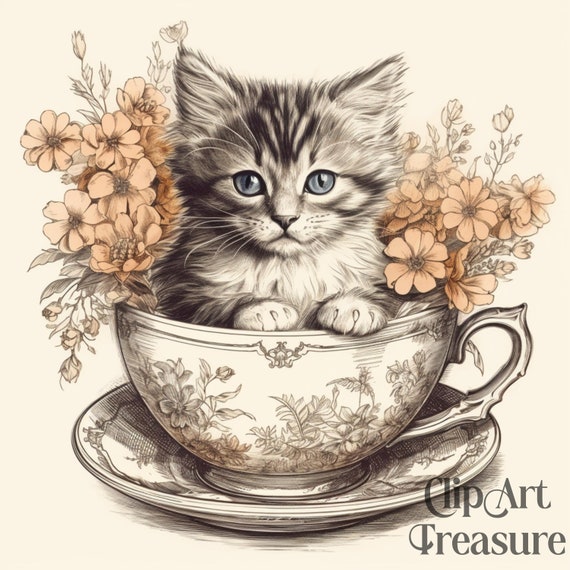The image showcases a detailed line drawing titled "Clip Art Treasure," featuring an endearing black and white kitten with pale blue eyes, nestled inside a large, ornate teacup. The small kitten, with its characteristic pencil-stroked fur, is poised with its paws on the rim of the soft off-white teacup, gazing directly at the viewer. The teacup, adorned with intricate floral and leafy designs in hues of gray and brown, sits atop a matching saucer. On either side of the kitten, delicate orange flowers with brown stems emerge from the teacup, adding a splash of color against the muted tones. The background includes additional flowers in shades ranging from yellowish-tan to gray, enhancing the overall charm of the scene.